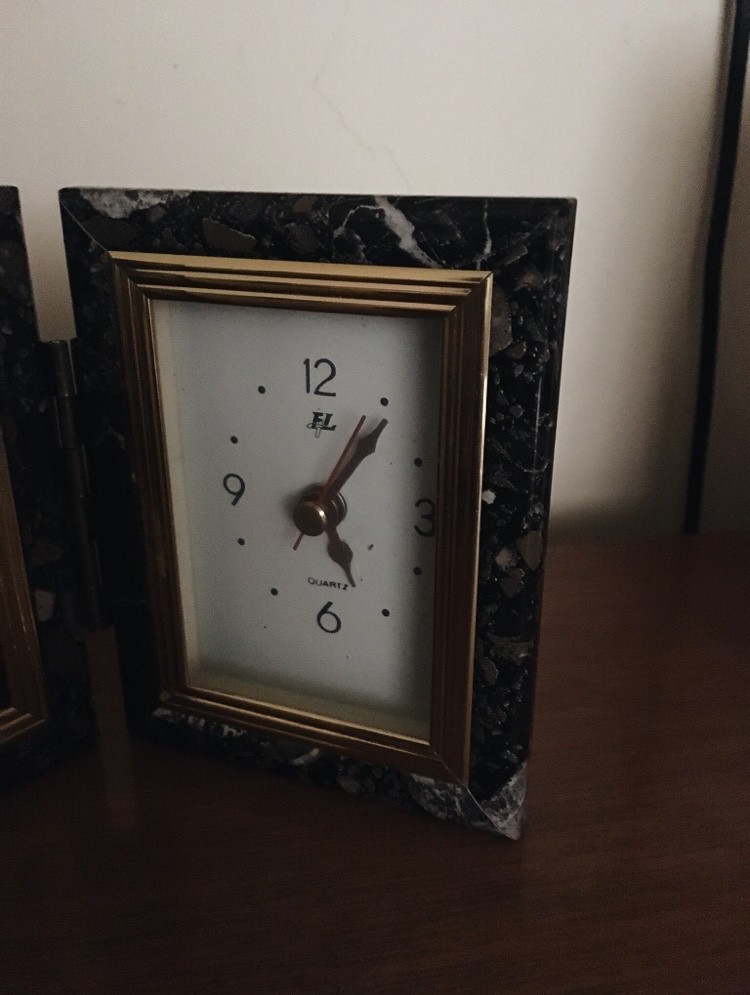The image depicts a close-up of a vintage-style alarm clock standing on a wooden nightstand against an off-white wall. The clock, slightly tilted with its left side higher than its right, features an ornate black and gray frame resembling marble, accented by a multi-layered gold bezel around the white clock face. The face shows the numbers 12, 3, 6, and 9, with dots marking the other hours, and it is equipped with three hands: a golden minute and hour hand, and a black second hand, indicating the time is approximately six minutes past five. Below the number 12, the letters "FL" are visible. To the right side of the image, a black electrical cord descends halfway down the wall, casting a gray shadow. On the left side, something dark and indistinct can be seen in the wood. Overall, the scene suggests a cozy, rustic setting with a hint of modern electronic influence.